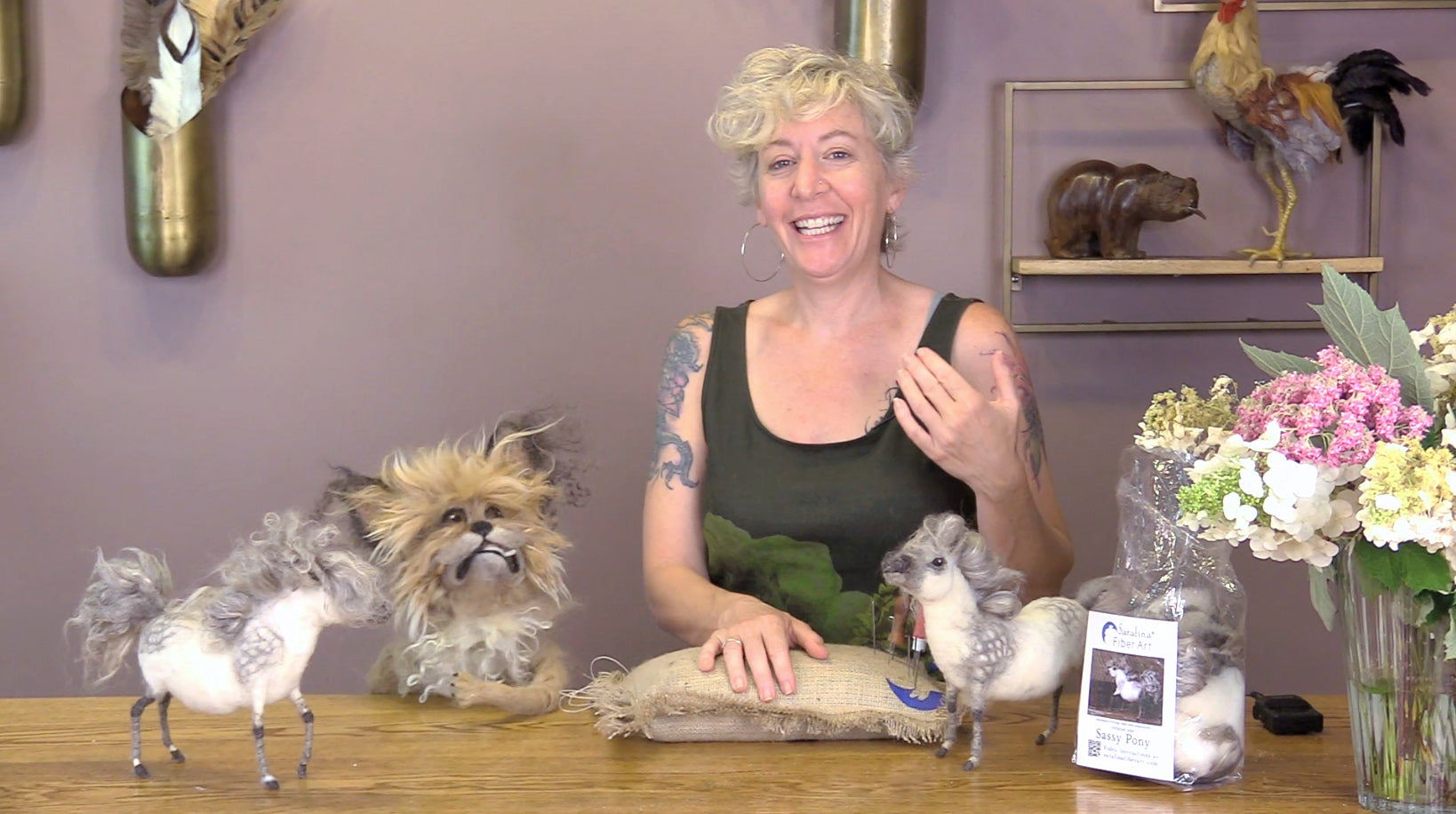In this photograph, a woman stands behind a table laden with intricately crafted animal figures. Smiling directly at the camera with her mouth open, she reveals both rows of teeth in a friendly expression. Her left hand is raised high above her t-shirt, while her right hand rests on a straw-colored, possibly textured pillow, which resembles burlap and might have sewing implements sticking out of it. Directly in front of her on the table, there is a small horse figure with white and gray fur, and another similar horse figure to its left. Both are detailed with actual fur, indicating they are likely handmade.

To the woman's right (left from the viewer's perspective) is a peculiar dog-like puppet with orange fur around the face and little black fur around the ear trims, its quirky expression adding a whimsical touch. Further to the right, a wooly unicorn puppet with white and gray fur stands on the table. Nearby, a plastic bag contains another one of these stuffed animals, hinting at more of her craftwork. A bouquet of flowers in a vase is situated at the bottom right corner of the image.

The background features a long wall adorned with what appears to be a wooden rooster and a bear, perhaps elements of her display. The overall setting suggests she is showcasing her handmade creations, which include these uniquely crafted animal figures.